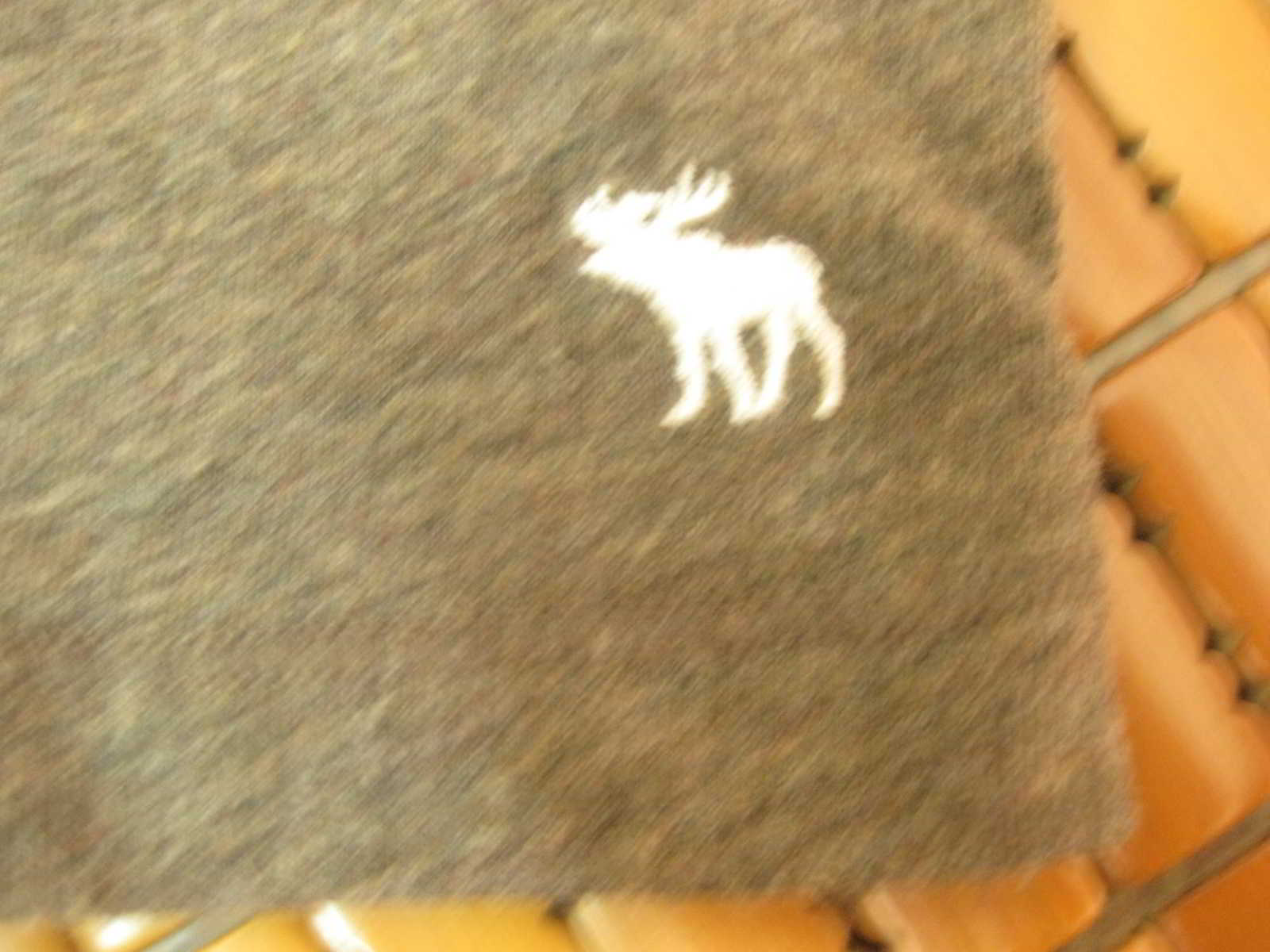This image features a detailed close-up of a medium gray fabric, possibly part of the sleeve of a shirt, intricately woven with white threads and specks, adding texture and depth to the material. Prominently stitched into the fabric is a white icon depicting a moose, characterized by its large, imposing stature and distinctive antlers. The moose stands firmly on all four legs, with its left antler prominently displayed. This antler, shaped like a long horn, branches into four prongs. The right antler is partially obscured and blends into the background, likely due to the perspective of the camera. This fabric rests atop an orangish-brown, tile-like surface, which appears to be a stitched-together background, providing a warm and contrasting foundation to the cooler tones of the gray fabric.